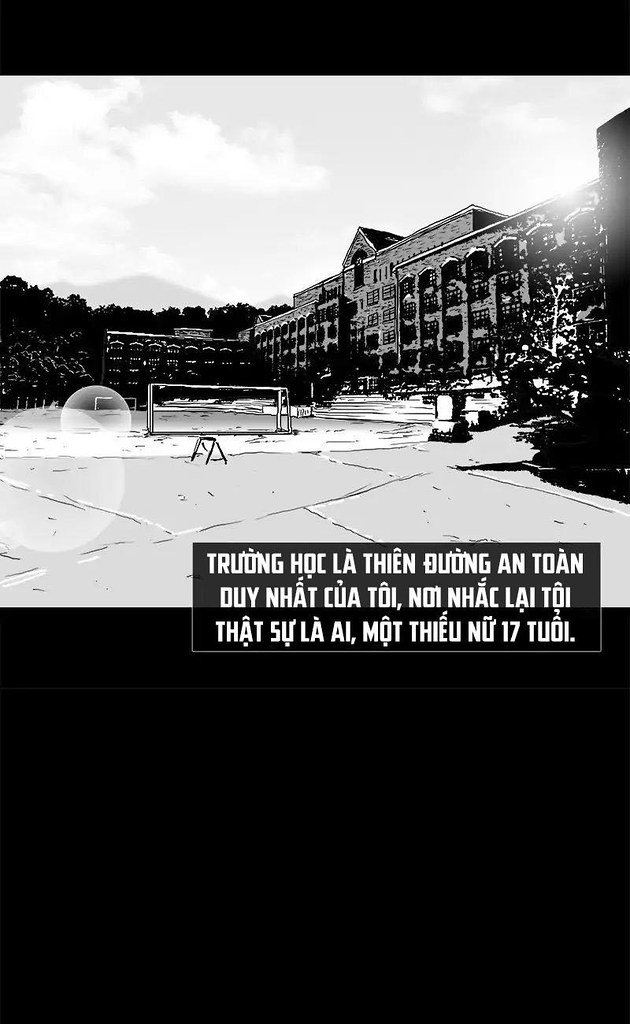This black-and-white, digitally generated image appears to depict a vintage scene. The layout features a thin black horizontal stripe at the top and a larger black rectangle at the bottom, framing the central vertical rectangular image. Dominating the right side of the image is a multi-storied institutional or college building, likely four or five floors high, characterized by numerous windows, a large central staircase, and a clock. On the left side of the image, a cluster of trees is visible with a faded mountain in the background under a predominantly white, cloudy sky. The foreground includes a spacious concrete walkway and what seems to be a playground or soccer field, complete with goalposts. In the bottom right corner, there's a black horizontal box with three lines of white text in an Asian language, concluding with the number 17.